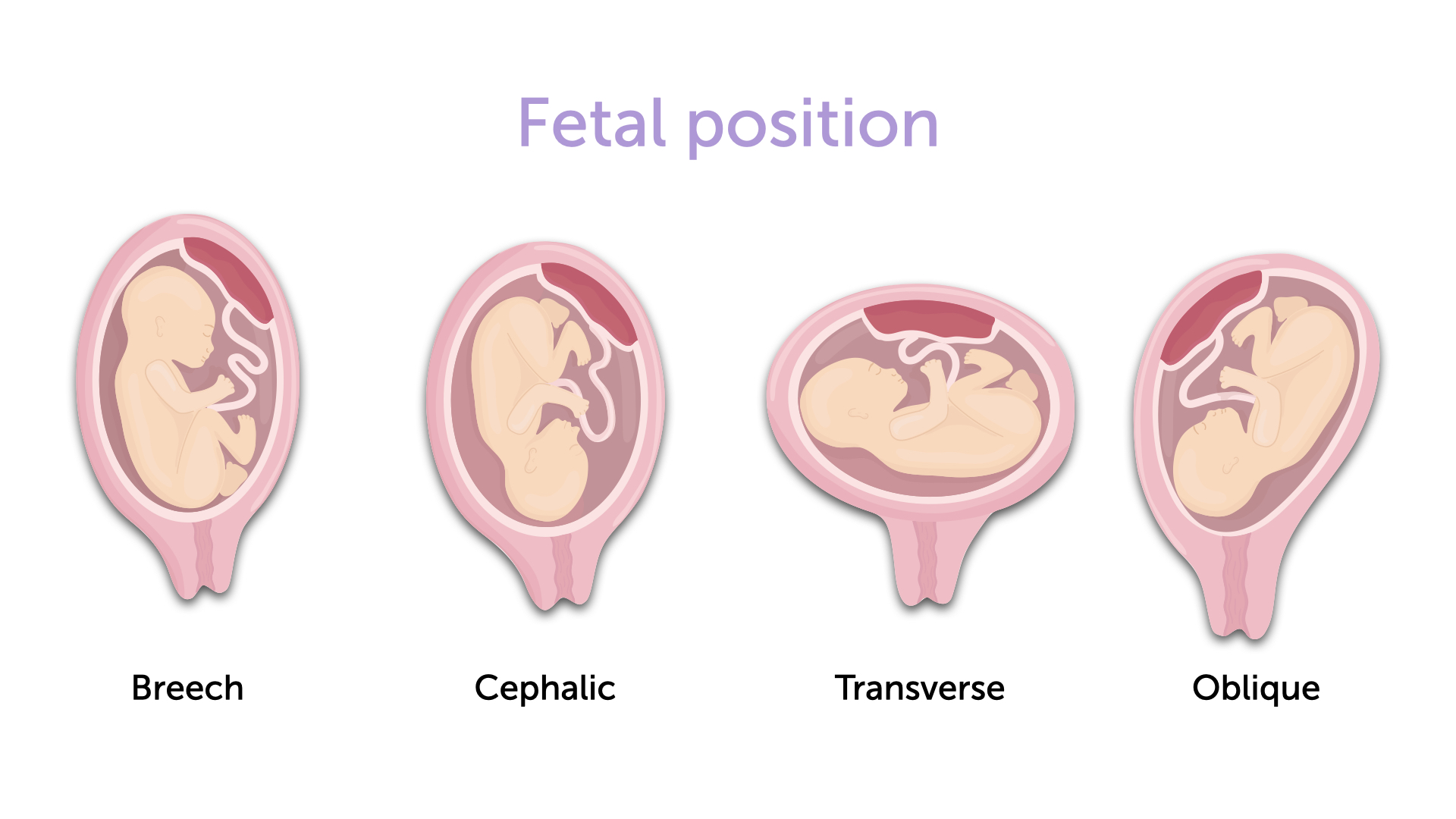The image is an artist's rendering titled "Fetal Position" that showcases four different fetal orientations within the womb, displayed in a clear, medically-informative manner often seen in a doctor's office. Each position is depicted within an oval, showing a baby in profile surrounded by the umbilical cord and amniotic fluid. 

1. **Breech**: The baby is upright, aligned with the natural egg shape of the womb.
2. **Cephalic** (spelled out clearly): The baby is upside down, positioned for birth.
3. **Transverse**: The baby lies horizontally across the womb.
4. **Oblique**: The baby rests at a diagonal angle.

The background is white, and the images are done in shades of pink and maroon, with the titles of each position written in black underneath the corresponding illustration. At the top, in purple text, the overall title "Fetal Position" is prominently displayed.